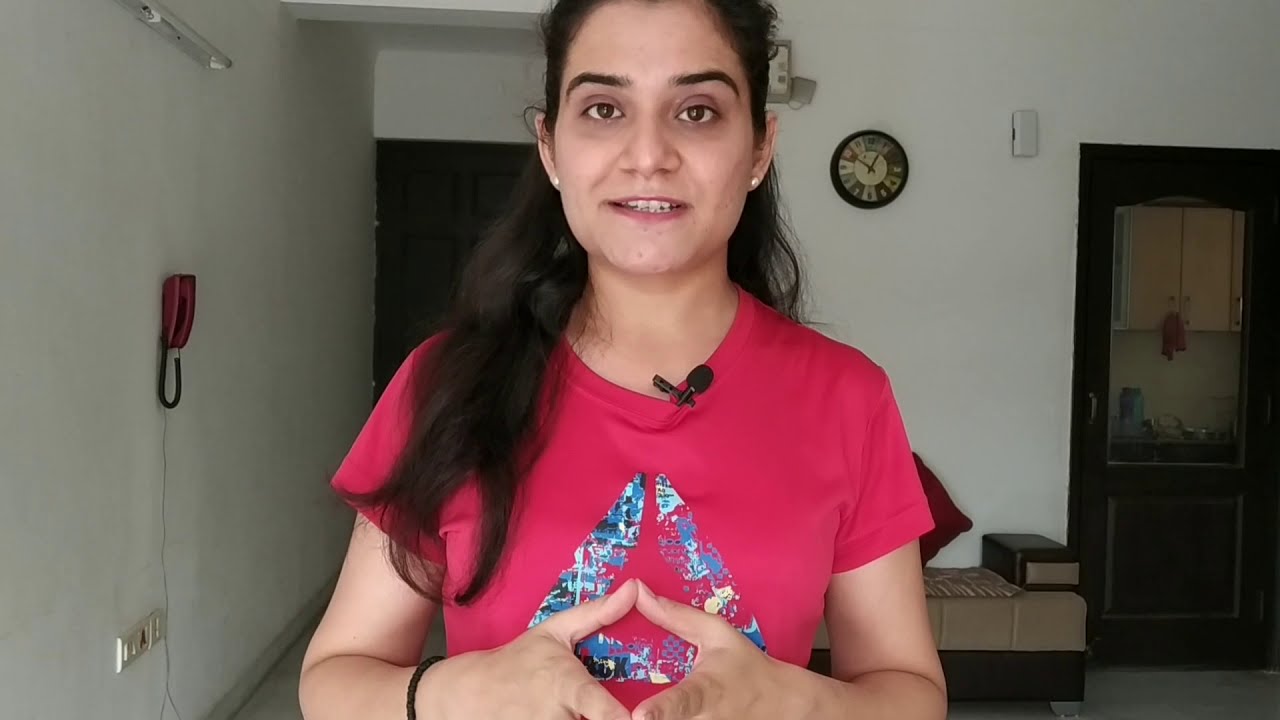In the image, a woman with long, dark brown hair and fair skin is captured mid-speech, with a small black microphone clipped to the collar of her dark pink t-shirt. She has her hands held together in front of her chest, forming a diamond shape with her thumbs and pointer fingers. She is looking directly at the camera with a half-smile, her eyes wide open. She wears white earrings and a brown beaded bracelet on her right wrist. The t-shirt features a triangle design in the center, composed of different shades of blue, yellow, and gray.

The setting appears to be the living room of an apartment or house, given the presence of white walls, a dark brown door on the far right, and another brown door on the left—possibly leading to a kitchen, as indicated by the glimpse of cabinets through a glass window. Behind her left shoulder is a clock with a black exterior, and over her right shoulder is a red phone with a black cord hanging on the wall. There is also a tan and dark brown sitting couch with a red pillow placed against one wall, and various outlets and horizontal fixtures can be seen. The woman is centered in the photograph, enhancing her prominence in the indoor scene.